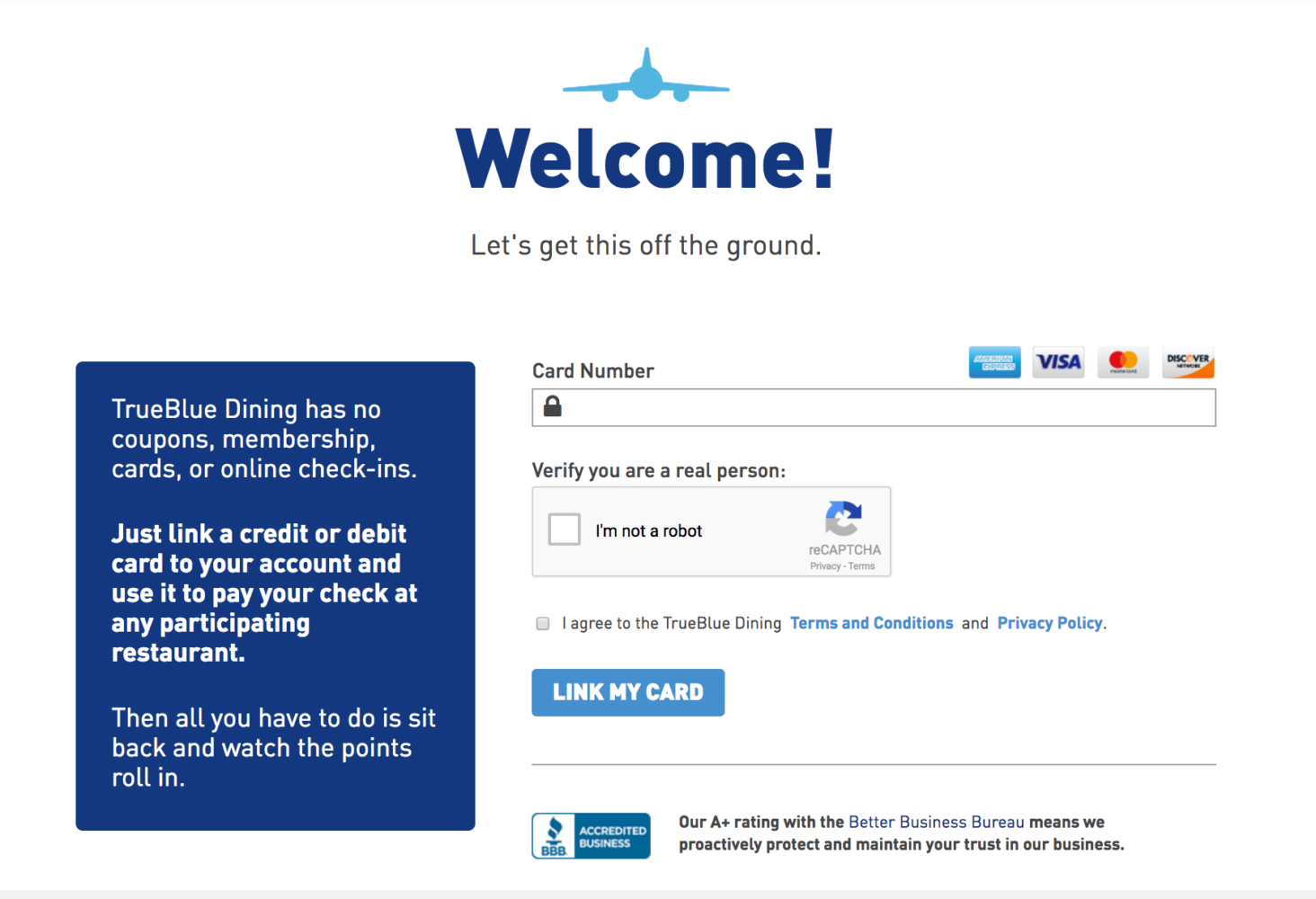The image depicts a computer screen displaying a registration page for a business named "True Blue Dining." The background of the screen is white. At the top center, there is a blue silhouette of an airplane, showing a central fuselage with wings extending to the left and right. Directly below the airplane graphic, large dark blue letters spell out "Welcome!" Beneath this, in smaller black letters, the text reads, "Let's get this off the ground."

On the left side of the page, a vertical blue rectangle contains white text explaining True Blue Dining's unique features: "True Blue Dining has no coupons, membership cards or online check-ins. Just link a credit or debit card to your account and use it to pay your check at any participating restaurant. Then all you have to do is sit back and watch the points roll in."

To the right of this blue rectangle, at the top, there is a labeled field to enter a card number. This field is situated above a lateral rectangle where users can input their information. To the left of this input box, a lock icon is displayed, signifying security. Above these fields, four colorful icons represent major credit cards: American Express, Visa, MasterCard, and Discover.

Below the card number field, the instruction "Verify you are a real person" appears, followed by a light gray lateral rectangle for CAPTCHA entry. Inside this rectangle, there is a white square labeled "I'm not a robot," accompanied by the CAPTCHA symbol and the text "reCAPTCHA privacy terms."

Further down, the caption states, "I agree to the True Blue Dining," followed by blue text linking to "terms and conditions" and "privacy policy." Below this agreement section sits a large blue rectangle with the words "Link My Card" in prominent white letters.

At the bottom of the screen, a thin gray line separates the content above from the section below, which features a lateral rectangle displaying the Better Business Bureau accredited business icon. To the right of this icon, black text highlights an A+ rating from Better Business Bureau, reassuring users, "Our A plus rating with Better Business Bureau means we proactively protect and maintain your trust in our business."